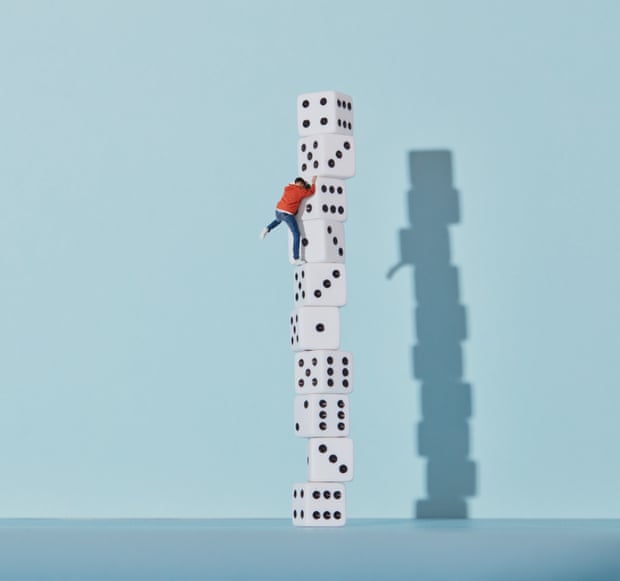The image features a precarious stack of 10 brightly colored dice, each rotated in varying directions, set against a light blue background that matches the darker blue surface they rest upon. The stark lighting casts a clear shadow of the stack to the right on the wall. Climbing this tower of dice is a small, detailed figure of a man. Dressed in a red hoodie, blue jeans, and white shoes, he is positioned near the top, around the seventh and eighth dice. His left foot is lifted in mid-climb, while his hands grasp onto the dice above him. Despite the tiny scale, his dark hair is distinguishable, though his facial features remain indistinct. The dice are oriented in such a way that starting from the bottom, they show combinations of 4 and 6, 3, 2 and 6, 5 and 6, 5 and 1, 5 and 3 (where the man’s foot is planted), 1 and 3, 6 and 4 (grasped by the man), 5 and 3, and capping off the tower at the top with 4 and 6. The scene creates a whimsical, larger-than-life adventure against a minimalist yet vivid backdrop.